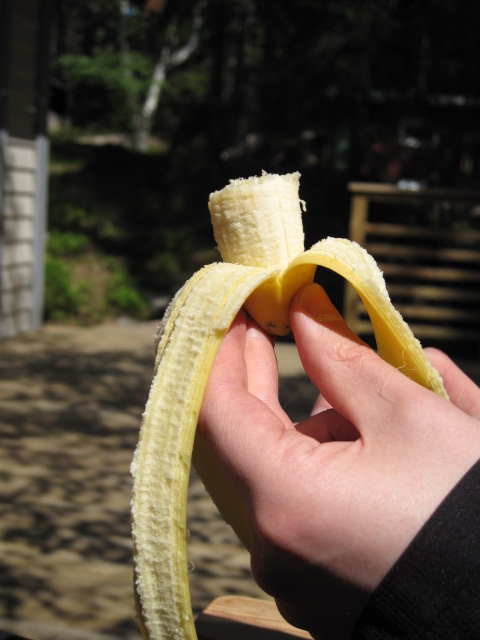A high-quality, portrait-oriented photograph captures an outstretched hand in the bottom right corner, holding a partially peeled banana. The hand, appearing to be of a fair-skinned individual, is positioned in a thumb opposition pattern, gripping the base of the banana. The banana peel is split open, with two sections flaring out to the left and right, just inside the thumb. Approximately two inches of the banana are visible, with about three-quarters of an inch within the peel and the remaining portion exposed, appearing to be either bitten or torn off. The backdrop includes a blurred, forest-like scene in the top half, with a blurry wooden railing to the right and shadowed concrete in the lower half, featuring the dappled shadows of tree leaves. The image's shallow depth of field emphasizes the hand and banana, maintaining sharp focus on these elements while keeping the background softly blurred.